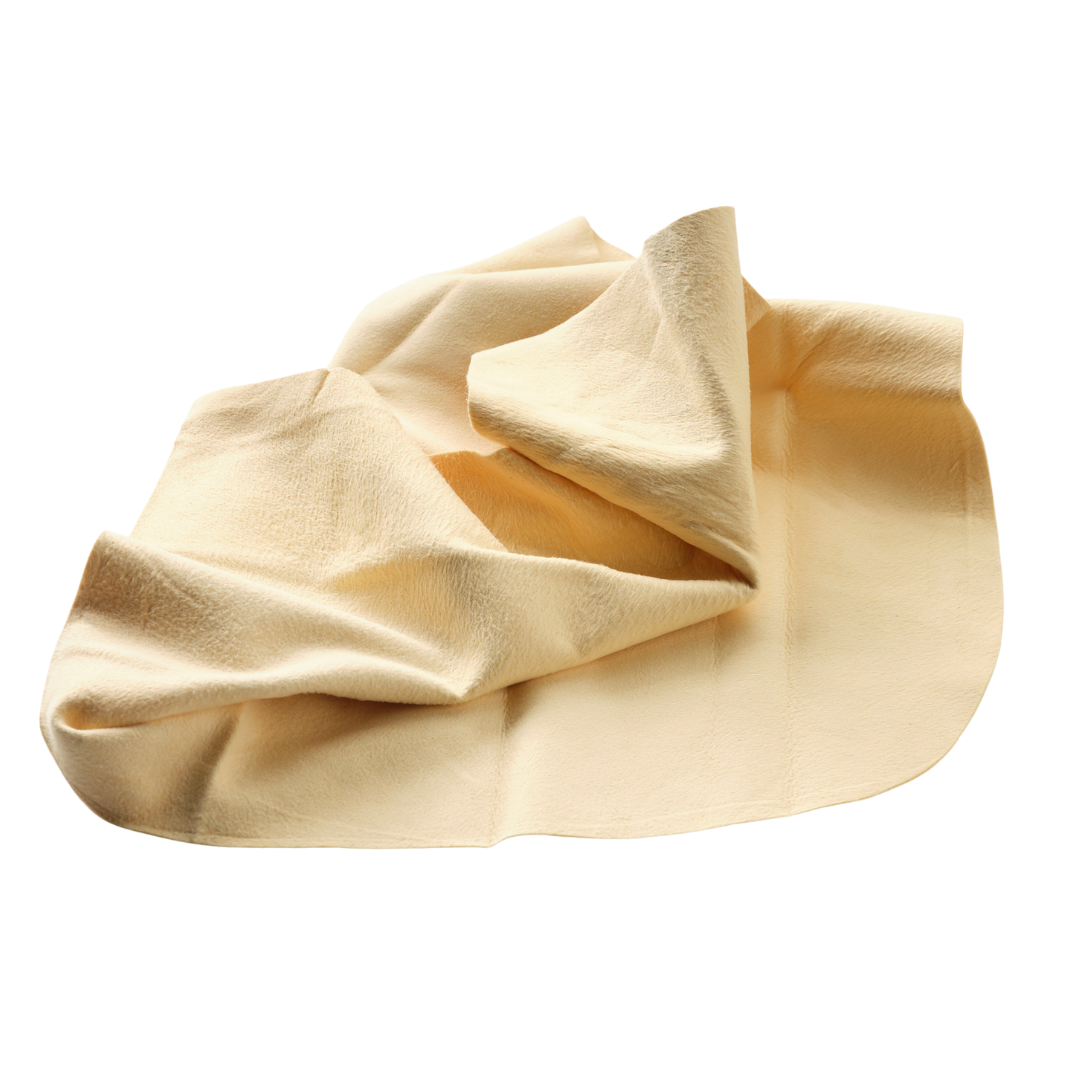This image is a detailed color photograph of a light beige to tan fabric, possibly resembling a chamois cloth, towel, or napkin, laid out on a stark white background. The cloth's texture is clearly visible, suggesting a suede-like material, potentially with visible fibers underneath. The fabric is arranged in an abstract manner with multiple folds: the upper left-hand corner is folded towards the center, and another section on the right is folded backward, creating darker tan shadows along the folds. The center of the image prominently displays the convergence of these folds, forming a visually striking shadowed area. Additionally, a small triangular fold appears towards the upper center of the cloth, adding to the overall abstract composition of the fabric.